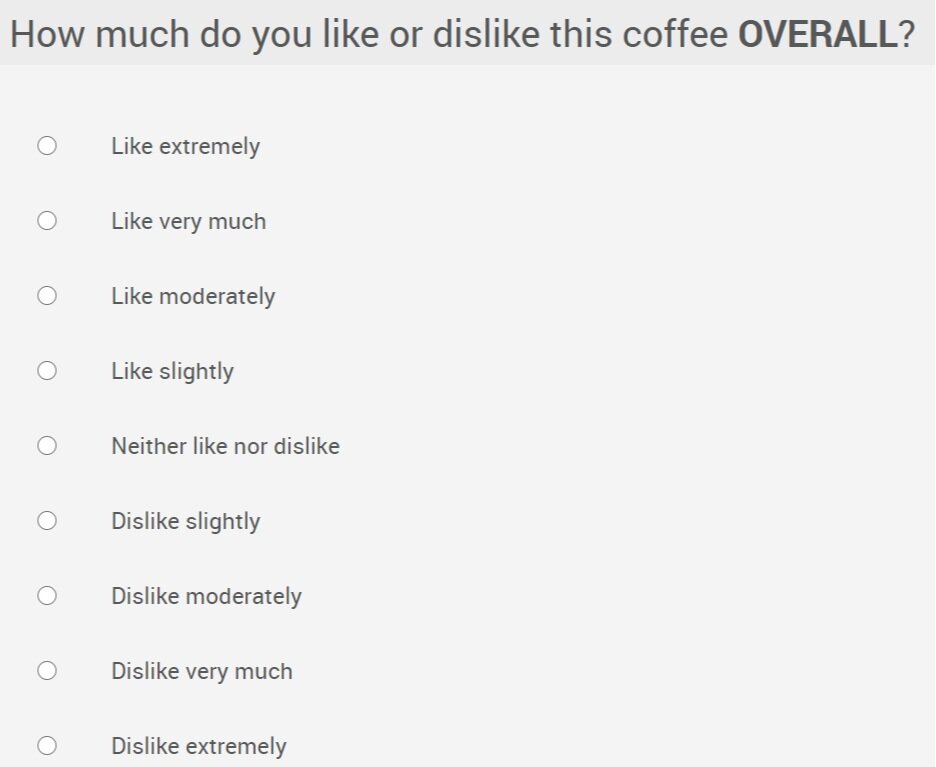Here is a detailed and cleaned-up caption for the image:

---

The screenshot showcases a survey question presented within a light gray box. At the top of the box, there is a slightly darker gray horizontal strip. In bold black text, the question asks, "How much do you like or dislike this coffee?" Beneath this, in all capital letters, the word "OVERALL" is prominently displayed. Below the question, there is a lighter gray area featuring a vertical list of multiple-choice options to gauge the user's preference. Each choice is accompanied by a white circle with a black outline for selection. The options range from "Like Extremely," "Like Very Much," "Like Moderately," "Like Slightly," "Neither Like or Dislike," "Dislike Slightly," "Dislike Moderately," "Dislike Very Much," to "Dislike Extremely." This gray box serves as a straightforward visual aid for rating coffee, providing clear and organized choices.